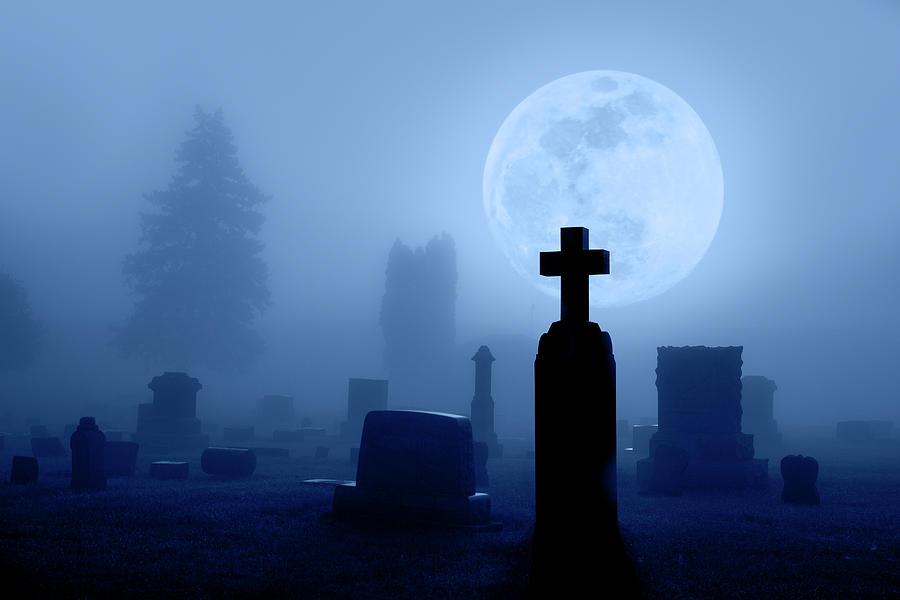The image depicts a fog-shrouded cemetery at night under a bright, full moon positioned in the top right-hand corner. The fog obscures much of the background, rendering the silhouettes of trees, including a prominent pine tree, blurred and indistinct. In the foreground, a tall, dark headstone with a cross atop stands out starkly. Surrounding this headstone are numerous other gravestones of various shapes and sizes, creating an assortment of small, medium, and large monuments. The thick fog blankets the ground, eliminating any visible grass and enhancing the eerie, ethereal atmosphere. The overall scene evokes a haunting, almost spectral ambiance, reminiscent of something out of a Halloween advertisement.